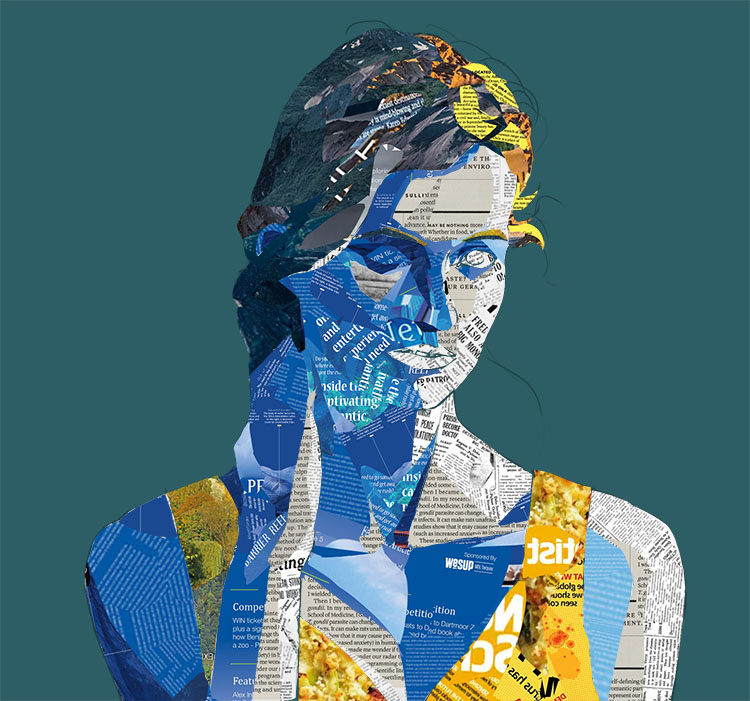This image showcases a vibrant and intricate craft piece. Set against a teal-blue background, it portrays the silhouette of a woman from her shoulders up, assembled entirely from various cuttings of newspapers, books, and magazines, giving it a collage-like appearance. The cuttings come in a spectrum of colors, including white, blue, yellow, and orange, with text in both black and white ink. The woman's hair, primarily dark with hints of blonde, and her face, partially obscured by one hand resting on her neck, add depth to the piece. She appears to be wearing a brown top with shoulder straps and no sleeves. The meticulous arrangement of text and images within the collage suggests either a highly sophisticated computer-generated design or an incredibly detailed handmade artwork. This blend of textual and visual elements creates an engaging and thought-provoking composition.